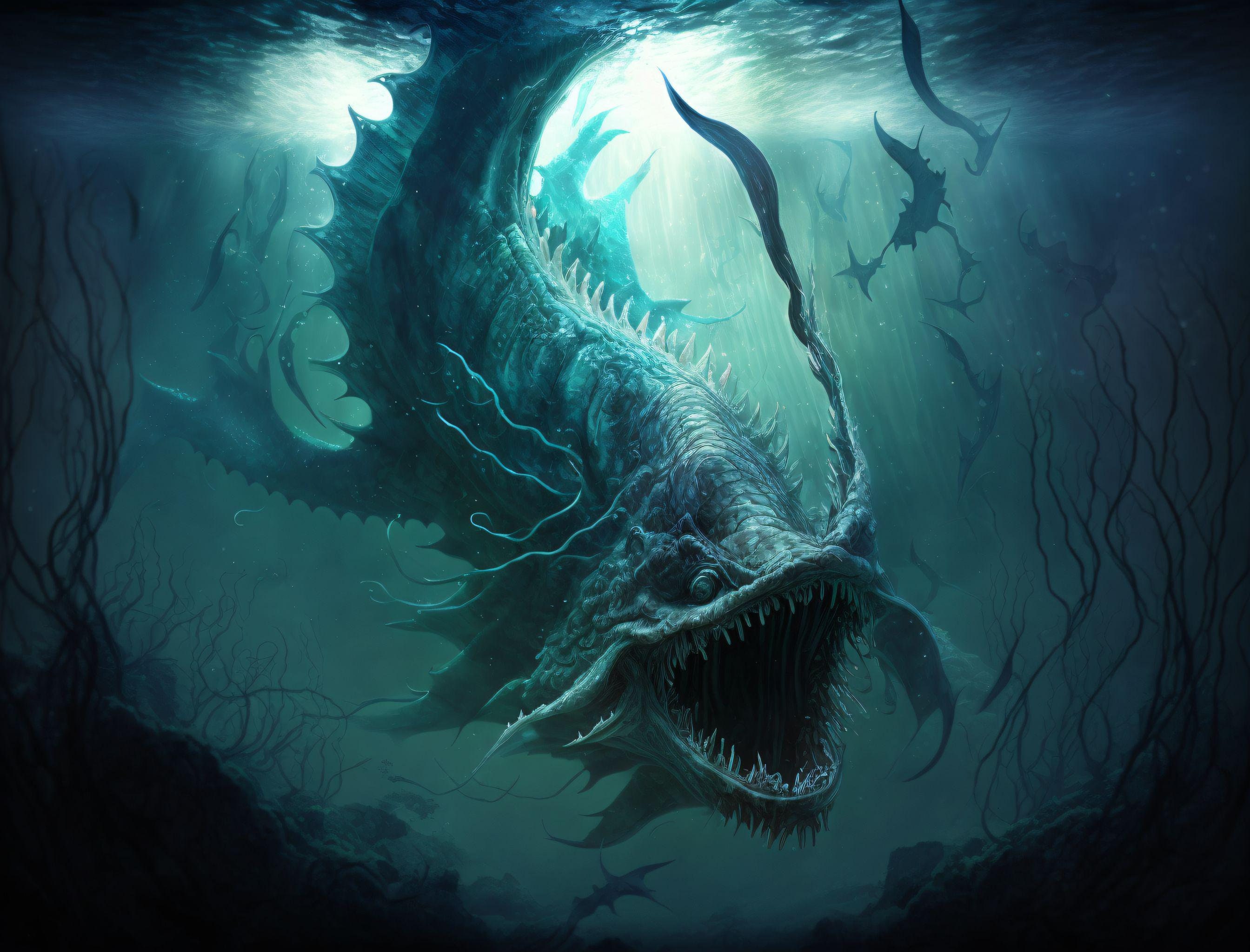This detailed digital art image portrays a haunting underwater scene dominated by a massive sea monster, reminiscent of mythical sea dragons or monstrous fish. This creature's body glistens with scales of blue and silvery hues, reflecting the greenish-blue tones of the surrounding water. Its form is adorned with sharp, thorn-like spikes and extensions running along its back and fins, giving it a menacing, almost otherworldly appearance. Its mouth gapes open, revealing rows of large, spiky teeth that add to its fearsome look.

The underwater environment is dark and eerie, with twisted, branch-like vegetation growing from the ocean floor and floating upwards toward the surface. Among these plants, smaller fish are scattered, further accentuating the sheer size and dominance of the sea monster. The visual elements of this digital painting combine to create a vivid and terrifying scene, with intricate details that capture the monstrous beauty of an underwater predator as it traverses its shadowy domain.